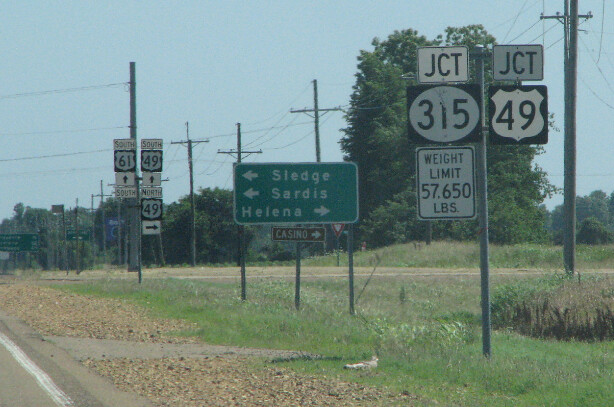The image captures a rural roadway scene under a clear blue sky with no clouds. The road runs along the left side of the image, with a gravel shoulder and a grassy central reservation. Several large, bushy green trees line the road, providing a natural backdrop. Several signs are present along the central reservation: the closest sign is green, indicating directions to the towns of Sledge and Sardis to the left, and Helena to the right. A smaller brown sign below it points to a casino on the right. Further along, another sign reads "Junction 315" and "Junction 49" with a weight limit of 57,650 pounds. In the background, a green sign directs "South 61" and "South 49" straight ahead and "North 49" to the right. Power lines run parallel to the road, adding to the rural setting. The area features tall prairie-style grass and a few more road signs, contributing to the comprehensive wayfinding system visible in this tranquil countryside vista.